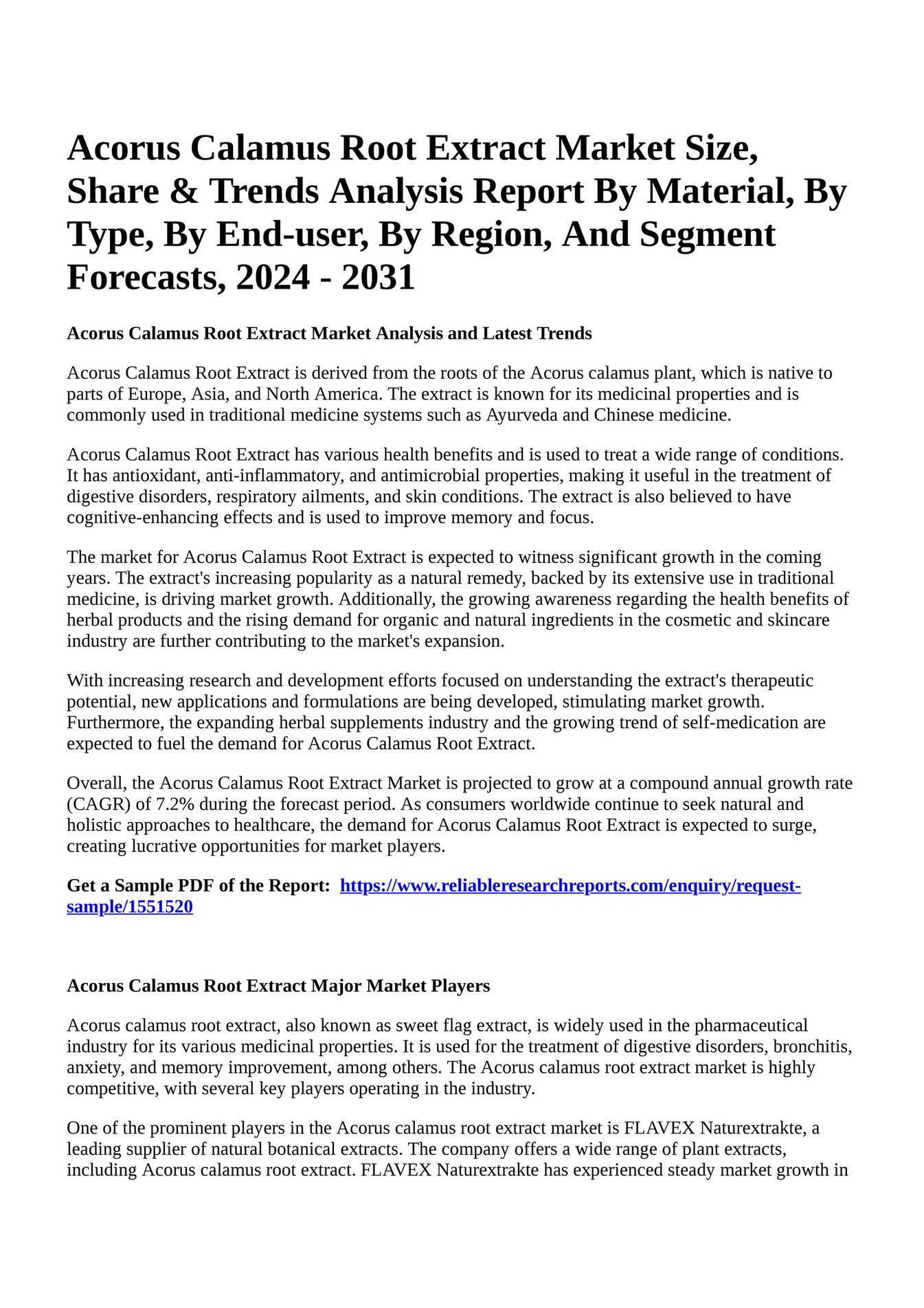The image features text from an article titled "Acorus Calamus Root Extract Market Size, Share, and Trends Analysis Report by Material, by Type, by End User, by Region, and Segment Forecasts 2024-2031," presented in large, bold, serif font. Below this main headline, a subheading reads "Acorus Calamus Root Extract Market Analysis and Latest Trends." The document provides a detailed analysis of Acorus calamus root extract, a substance derived from the roots of the Acorus calamus plant, which is native to Europe, Asia, and North America. The extract is known for its medicinal properties and is commonly used in traditional medicine systems like Ayurveda and Chinese medicine due to its antioxidant, anti-inflammatory, and antimicrobial properties. The report discusses its health benefits in treating conditions such as digestive disorders, respiratory ailments, and skin conditions. The article is structured with multiple sections, including a call to action in bold text for obtaining a sample PDF of the report, along with a hyperlink. Another section titled "Acorus Calamus Root Extract Major Market Players" elaborates on key pharmaceutical industries involved in the market.